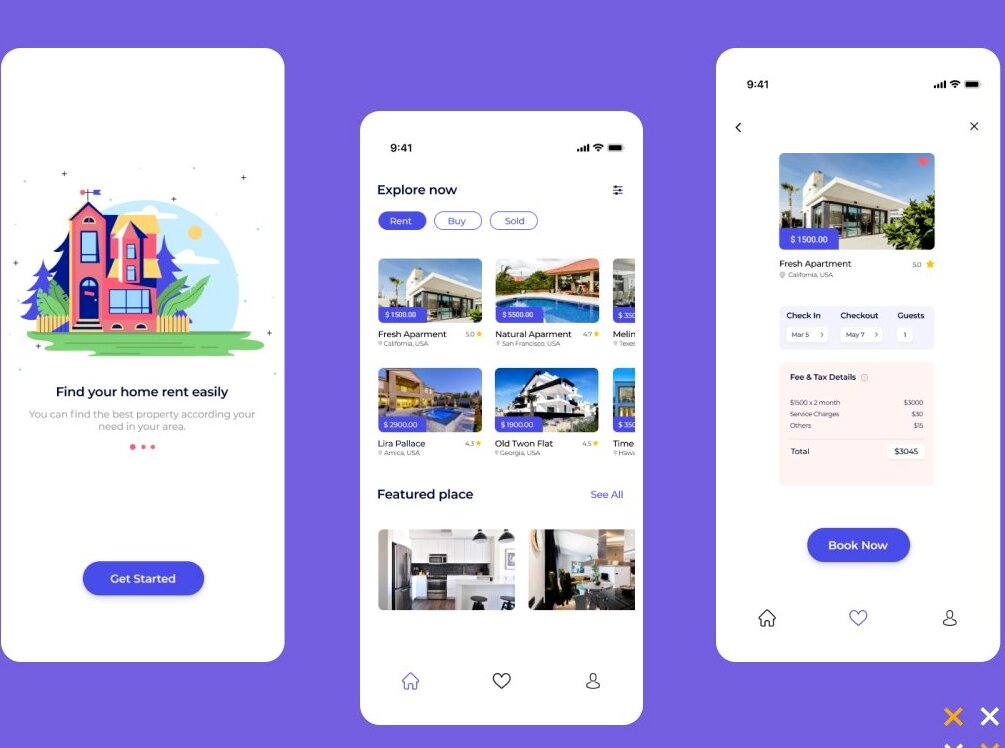Three screenshots showcase different features of a home rental application. The first screenshot emphasizes the ease of finding rental properties with the headline, "Find Your Home Rent Easily," followed by "Get Started." This is visually framed at the bottom with a prominent blue rectangle button labeled "Explore Now." The options "Rent," "Buy," and "Sold" are presented in clickable rectangles, with "Rent" highlighted in blue, indicating it is currently selected. Beneath are several thumbnail images of homes labeled as "Featured Places" and a prompt to "See All" for additional listings.

The second screenshot continues with more images of homes, again categorized under "Featured Places," though details are not fully clear in this summary.

The third screenshot, showing the time as 9:41, features a detailed listing for a "Fresh Apartment." It provides options to select check-in and check-out dates—shown as March 5th and May 7th, respectively—and accommodates one guest. A prominent blue rectangle button at the bottom invites users to "Book Now."

This detailed visual walkthrough highlights key functionalities and user interface elements of the app, designed to simplify the process of finding and booking rental properties.